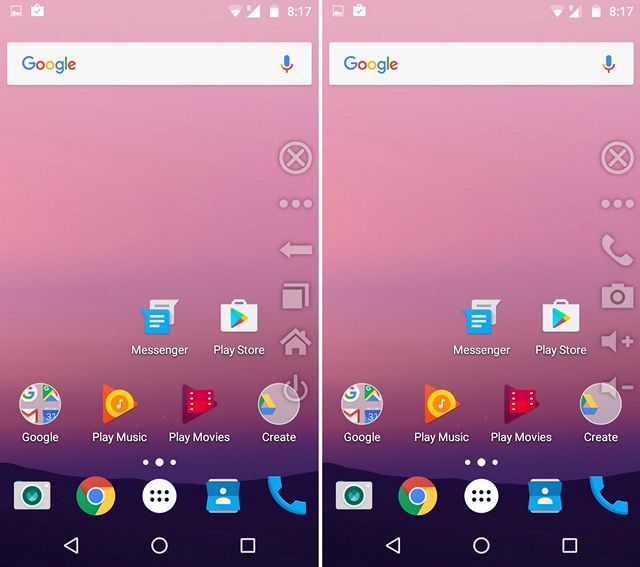The image displays two cellphone screens side by side. The background gradient starts with a dark blue, almost black hue at the bottom where stylized hills are depicted. This dark blue gradually transitions into a rich purple, which then blends into a deep mauve color. As the gradient continues upward, the colors become lighter until it culminates at the top with a soft pink shade.

At the top of the screens, standard status icons are visible, including cellular signal bars, Wi-Fi signal bars, and a mostly charged battery icon. The time displayed is 8:17 AM. Just below these icons is a Google search bar.

On the right side of the screens, several icons and symbols appear, including an 'X' within a circle, three vertically aligned dots, a back arrow, a white square with a line on the top right corner (possibly the copy icon), a house icon representing the home button, and a power symbol.

The screens are populated with various app icons. Among these are icons for messaging, the Play Store, Google search, text messaging, Play Music, Play Movies, an app named "Create", phone calls, navigation, the camera, and Google Assistant. There are also three dots arranged vertically in two rows within a white circle, an icon that resembles contacts, and another for the phone app again.

The icons on the right screen appear mostly in a translucent white color, while the rest of the icons maintain their standard colors such as red, yellow, orange, blue, green, black, white, and gray.